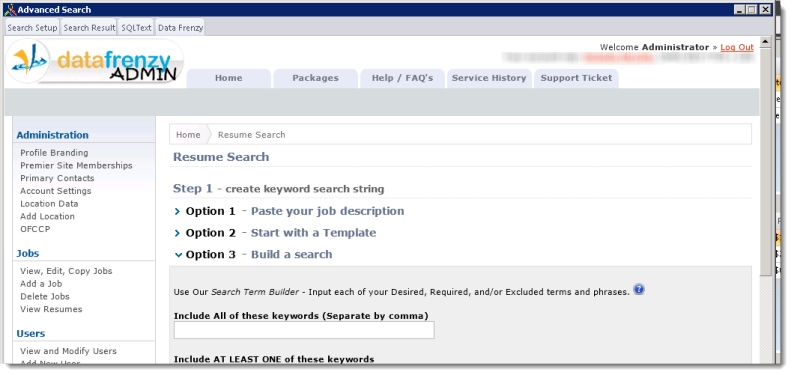**Detailed Description of the Website Interface:**

The screenshot showcases a website interface designed for advanced search functionality. 

- **Top Left Corner:** The phrase "Advanced Search" is prominently displayed, indicating the primary feature of the page. Below it, several link options are listed in the following order: 'Search Setup,' 'Search Result,' 'SQL Text,' and 'Data Frenzy.' A small circular icon labeled 'Data Frenzy Admin' follows, with 'Data' in yellow, 'Frenzy' in blue, and 'Admin' in black.

- **Navigation Tabs:** Adjacent to this section, several navigation tabs are aligned horizontally. They include: 'Home,' 'Packages,' 'Help/FAQs,' 'Service History,' and 'Support Ticket.'

- **Top Right Corner:** The interface greets the user with "Welcome Administrator," followed by a 'Log Out' button.

- **Left Sidebar:** Displayed vertically, the left sidebar features the following categories:
  - **Administration (in blue):** Under this heading, several sub-options are listed in black: 'Profile Branding,' 'Premier Site Memberships,' 'Primary Contacts,' 'Account Settings,' 'Location Data,' 'Add Location,' and 'OFCCP.'
  - **Jobs (in black):** This category lists options like 'View, Edit, Copy Jobs,' 'Add a Job,' 'Delete Jobs,' and 'View Resumes.'
  - **Users (in blue):** The final category includes the option 'View and Modify Users.'

- **Main Body:** The central part of the page features a structured layout:
  - A box labeled 'Home and Resume Search' followed by 'Resume Search.'
  - Steps for conducting a resume search:
    - **Step One:** 'Create Keyword Search String,' accompanied by two blue arrows pointing right and one blue arrow pointing down.
    - Users can choose from three options:
      - **Option 1:** Paste your job description.
      - **Option 2:** Start with a template.
      - **Option 3:** Build a search.

This detailed description highlights the structured and user-friendly design of the interface, aiding users in navigating through various advanced search functionalities.